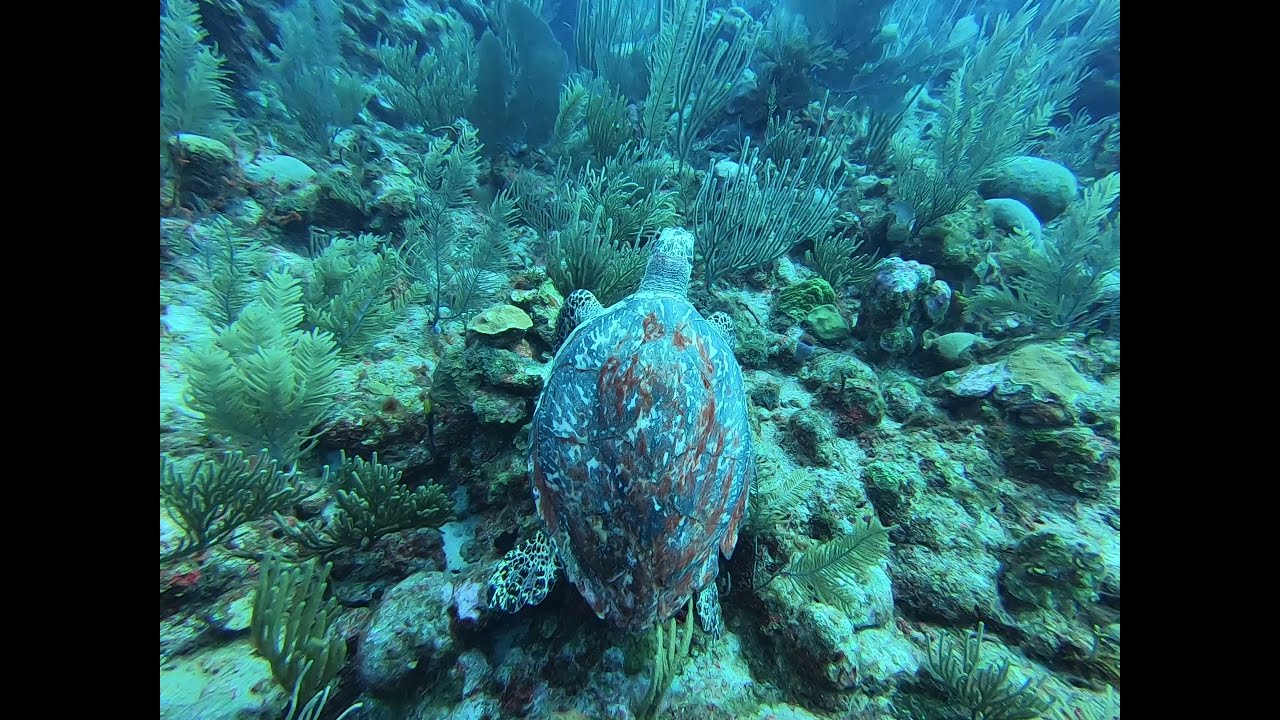In an underwater scene with a greenish-blue tint, a turtle with flat, thin-like legs takes center stage. It swims upwards in the image, revealing a dark gray shell adorned with white splotches and various brown spots. The turtle's head and four fins are visible, and it appears to be grazing or cruising over a seabed rich with sea life. Below the turtle, smooth round rocks covered with white spots and fern-like green plants are scattered across a white sandy ground. The underwater landscape extends as far as the eye can see, filled with coral and seaweed, giving the impression of a vast ocean or sea. Notably, there is some unidentified debris, possibly ocean-going trash, underneath the turtle's back left fin. The image is framed by two rectangular black bars on either side, adding to the underwater ambiance of the photograph.